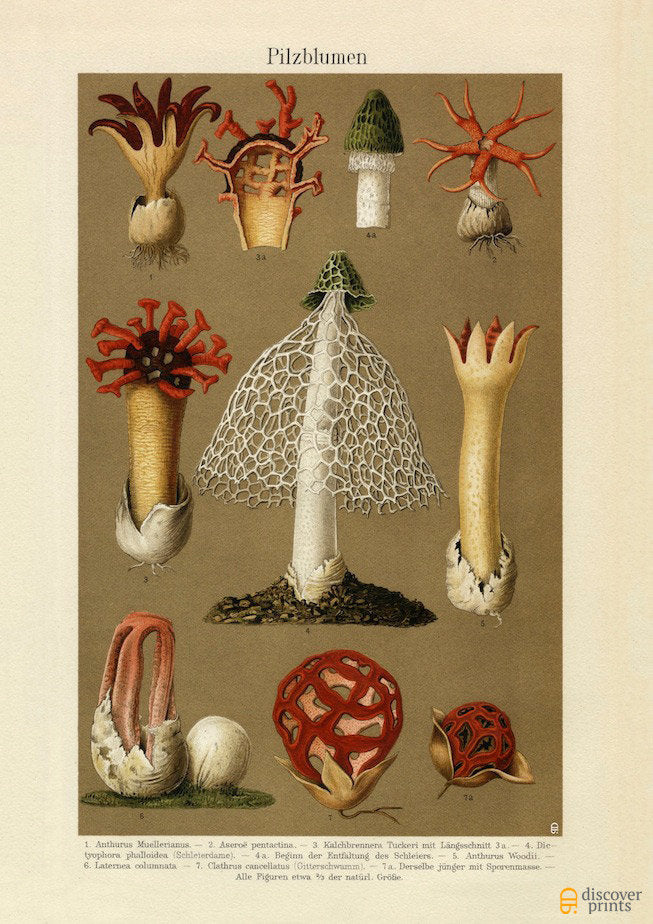The image is a detailed botanical chart titled "Pilz Blumen," displaying an array of otherworldly, alien-like fungi organized in three rows against a light tan mortar backdrop. The top row contains four distinct mushrooms, the second row three, and the last row also three, totaling ten peculiar and varied fungi. These mushrooms are depicted with unusual and intricate details, making them appear almost surreal. Notably, the central and largest mushroom features a white stalk with an umbrella-like cap perforated with numerous holes, while a smaller, similarly shaped green mushroom sits above it. Each fungus is accompanied by a name, likely in Latin, although the text is too small to be legible. Surrounding the green field of the chart is a thick white border, and in the bottom right corner, an orange pill-shaped logo with the words "Discover Prints for the Gangai" is visible just outside the frame, possibly indicating the source or theme of the chart.